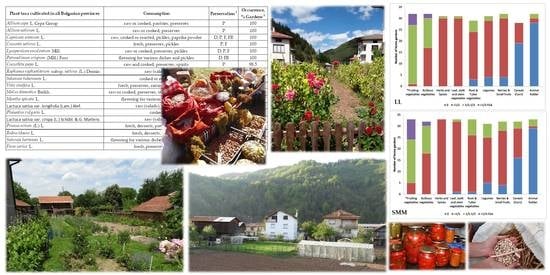The image is a horizontally rectangular collage predominantly made up of various smaller full-color photographs, tables, and bar graphs. The photographs, either square or rectangular, depict outdoor scenes mainly centered on nature and farm life. These include gardens, fields of flowers, farms, and homes, with one photo featuring a mountain, trees, and white buildings. In the lower right-hand corner, there is a detailed picture of jars containing a red substance, potentially canned tomatoes, next to another showing hands scooping grain from a white sack. 

The upper left corner contains a block of text that is too small to read, while the upper right corner features a pair of multicolored bar graphs (in red, green, and blue), also unreadable due to the fine print. Additionally, there’s a white table with black text and columns situated in the top half of the image, but it is similarly difficult to decipher. Overall, this collage appears to be an informational chart, likely conveying data about the farming area depicted in the photographs.